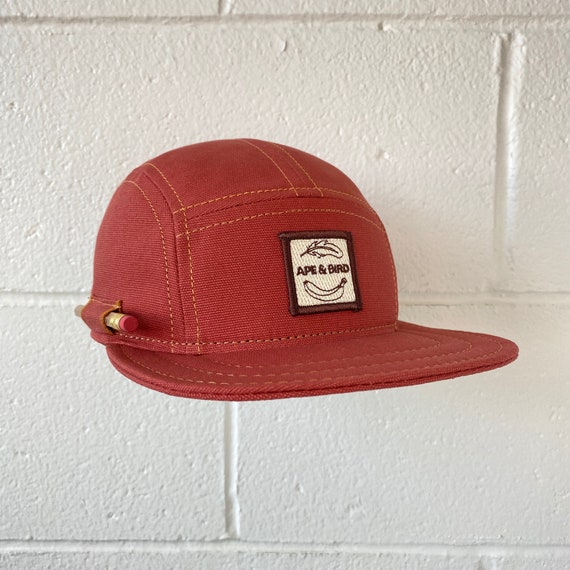This image features a unique burgundy corduroy ball cap, prominently displayed in front of a white cinder block wall reminiscent of school hallways. The cap stands out with its flatter, wider brim and an unconventional rounded style. A notable detail is the pencil holder loop situated above the ear on the left side, illustrated by a pencil inserted into it. At the center of the cap is a square logo patch with a dark brown border and a white background, showcasing intricate embroidery that reads "ape and bird." The logo is further adorned with a green leaf above the text and a yellow banana below it, all stitched with orange thread. The cap appears to be suspended in midair, adding an intriguing visual element to the advertisement-like presentation.